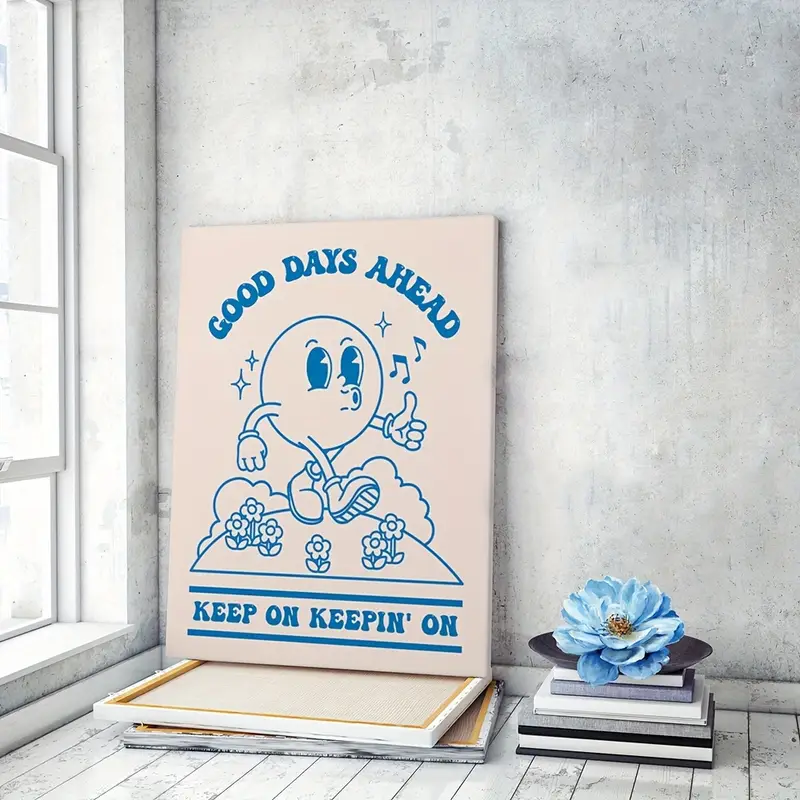The image depicts a corner of a room with a distinctly monochromatic color scheme, dominated by shades of gray, white, and black. The walls, which have a concrete-like texture, and the gray-washed wood plank flooring, give the room a somber, almost bleak appearance. On the left side of the image, a large window with a gray outline extends from the floor to the upper part of the scene, reminiscent of a classic New York apartment window.

Central to the image is a canvas leaning against the wall. The canvas is cream-colored with blue graphics and text. At the top of the artwork, it reads "Good days ahead," and at the bottom, "keep on keeping on." In the middle, there is a simple line drawing of a small, round character, humanoid in appearance with eyes, a mouth, and hands. The character appears to be whistling, as indicated by music notes drifting from its pursed lips, and is walking among blue sunflowers and other shrubberies. This character's environment on the canvas seems to depict a curved ground, giving a whimsical touch to the otherwise stark setting.

The canvas rests atop two other upside-down canvases, obscuring their content. To the right, there is a neat stack of four or five books or journals, also in the gray, white, and black color palette, with one having a bluish-gray hue. Sitting atop the books is a vivid blue flower with light blue petals and a yellow center, likely resting on a plate. The flower stands out sharply against the grayscale background, adding a pop of color that contrasts with the otherwise desaturated theme of the room.